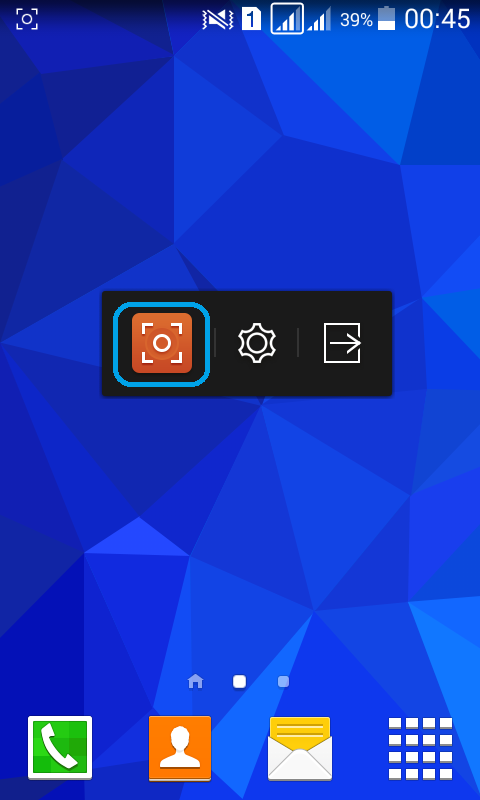A screen capture of a smartphone's interface, possibly from Vodafone, typical of devices from Asia or India. The display shows the time as 00:45 (or 12:45 AM), with the battery level at 39% and three out of four bars for network reception. The speaker is muted. Central to the screen are three interactive icons: on the right, a door with an arrow likely indicating a 'return' function; in the middle, a cogwheel representing 'settings'; and on the left, a selected icon highlighted with a border, depicting a red square with intricate angles inside and a central circle.